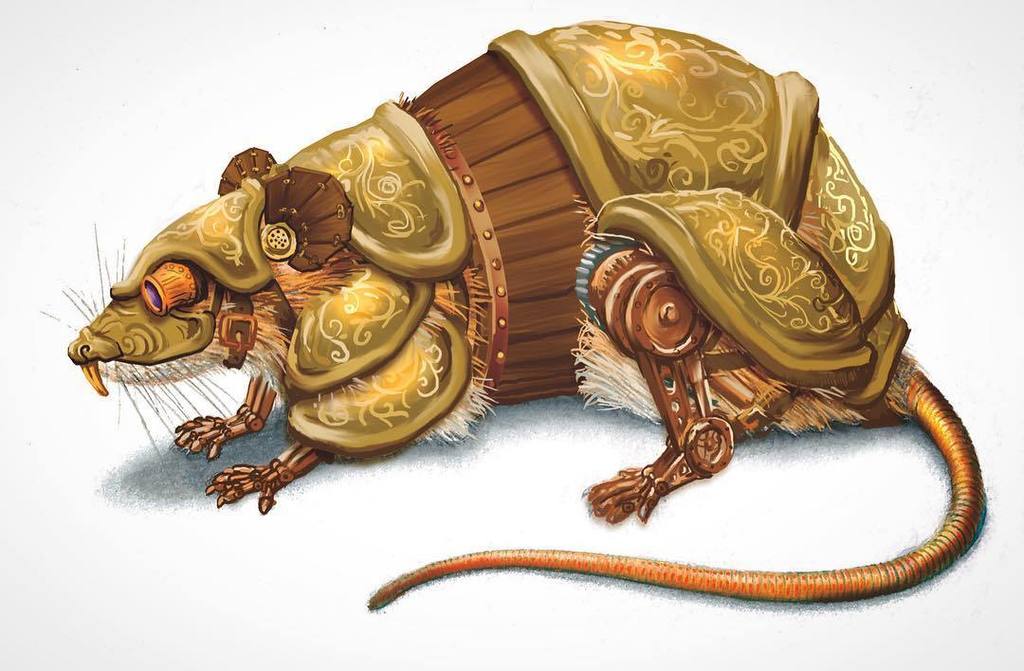This detailed, hand-drawn image depicts a steampunk-style rat displayed in a larger format. The rat is intricately designed with a blend of medieval and futuristic elements. Its head, covered in ornate, gold armor with intricate swirls and detailing, features a golden eye lens or goggle and a conspicuous gold tooth. The armor extends to its body, which includes wooden planks forming its torso and ears, and appears to have little speaker-like devices where its ear holes would be. The rat's mechanical arms and legs are made of metal, and its long tail resembles copper coils, twisted into the beginning shape of a question mark. Enhancing its steampunk aesthetic, the rat has a collar made of chains and sports corkscrew-shaped eyes, combining elements of fabrication through nuts, bolts, and screws that suggest a craftsman's handiwork.